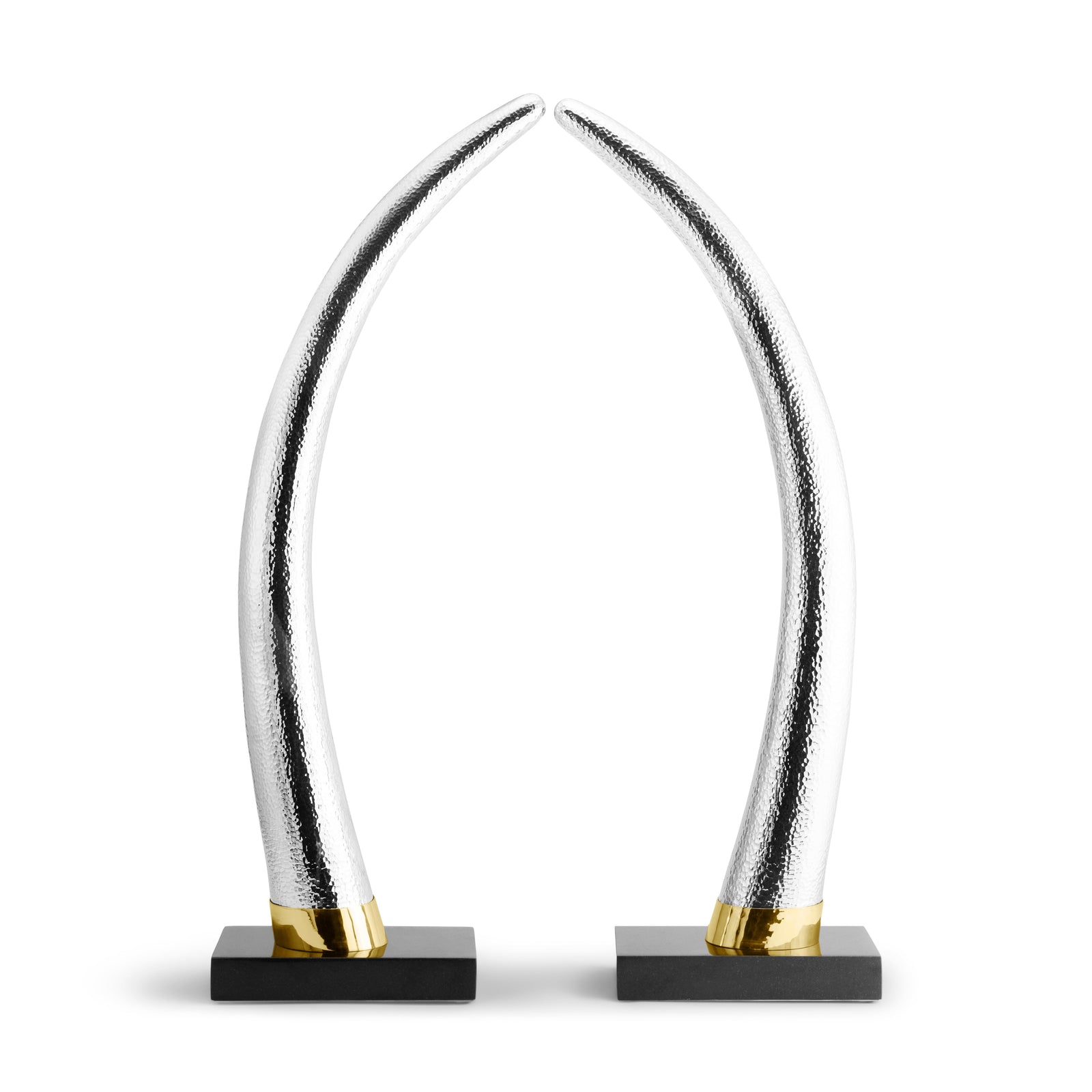The photograph captures a striking art piece displayed against a stark white background, enhancing its vibrant details. Centered on a dark gray, rectangular block, the sculpture consists of two identical, silvery-white horns with a lustrous, textured surface, forming an arch as they curve towards each other. The horns, resembling elegant tusks, have a distinct black section in the center and feature golden cuffs at their bases, adding a touch of warmth to their metallic sheen. This intricate design appears both functional and decorative, potentially serving as an elaborate paperweight or simply a captivating sculpture.